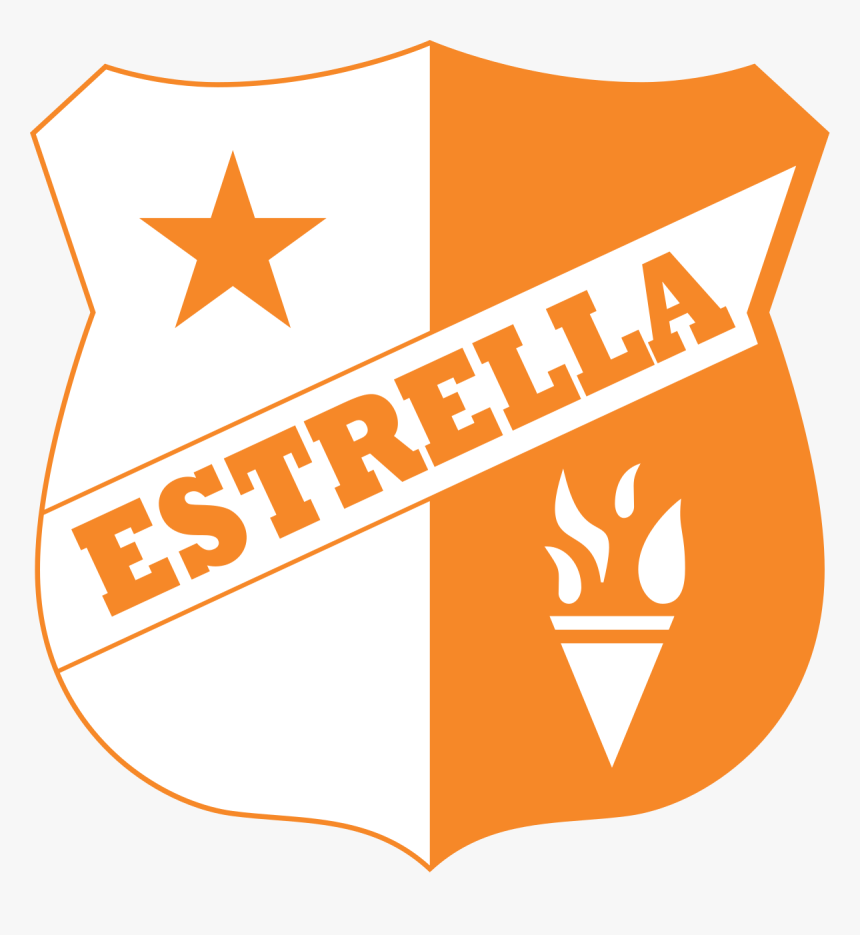The image is a detailed computer-generated logo or badge set against a solid light gray background. The badge, which occupies most of the space, features a unique shape that starts with two curved lines at the top, transitioning into angled edges, and rounds out down the sides, finally meeting at a pointed tip at the bottom. The badge is equally divided into two vertical halves: the left half is white, adorned with an orange star in its upper section, while the right half is orange, featuring a white upside-down triangle with a line above it and flame-like details at the bottom. Diagonally across the badge runs a white sash bearing the word "Estrella" in capital orange letters. The letters start with "E" at the lower left section and end with "A" at the upper right section of the badge. The design combines elements suggestive of a family crest or a sports team logo, showcasing a minimalistic yet striking use of the colors orange and white.